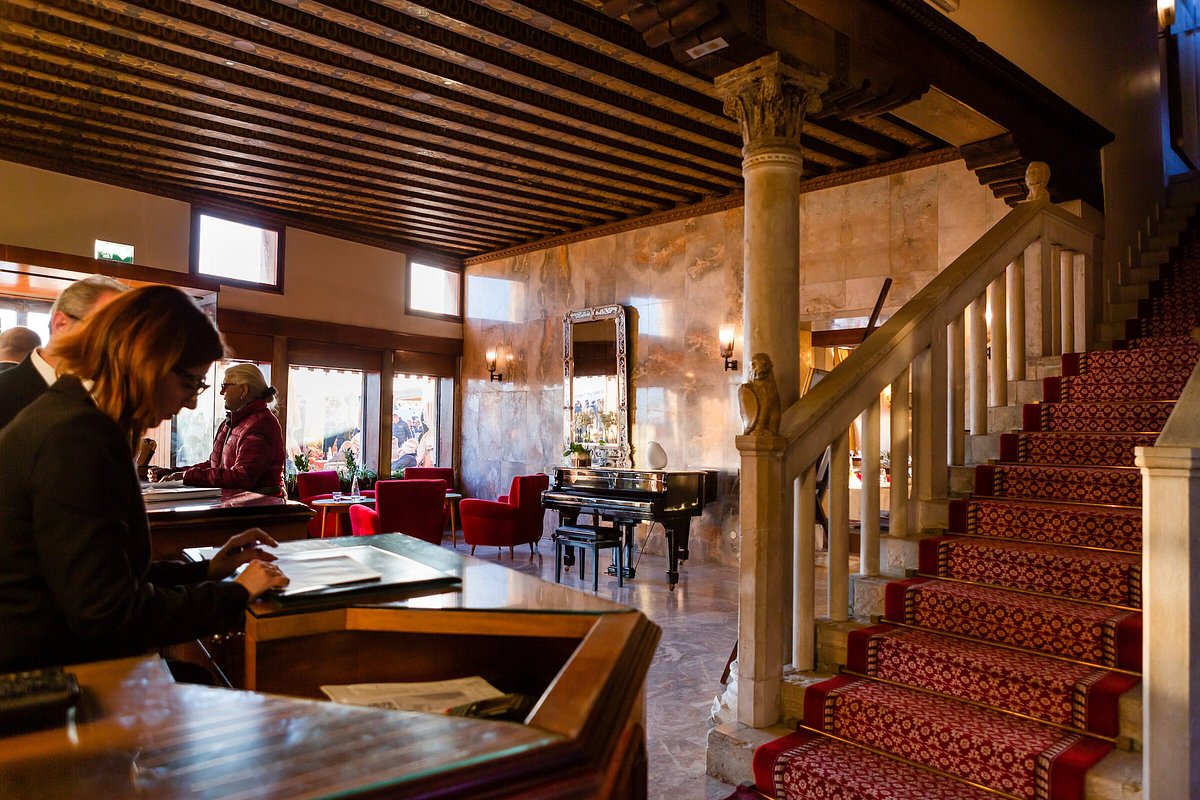The image depicts the interior of an elegant, old-fashioned hotel lobby, bathed in warm hues. A wooden counter with a drop-down section is situated on the left, attended by a woman with shoulder-length hair, glasses, and a dark shirt, engrossed in some papers. Behind her, the top part of a man's head is visible. The space is adorned with dark wood beams spanning the ceiling, complementing the marble walls and floor. To the left are high, sunlit windows that provide a view outside, alongside red chairs arranged around a table. A large mirror hangs on the marble wall near a grand black piano. On the right, a gold-accented staircase with a patterned red carpet runner ascends to the upper floor. The overall atmosphere is one of timeless sophistication and classic design.